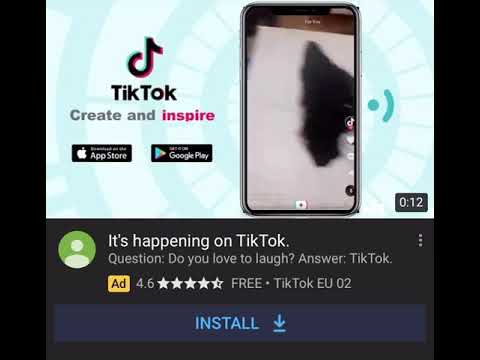This image is a rectangular screenshot with a predominantly solid black background encompassing the bottom, left, and right edges. At the top, a light blue and white geometric design serves as a backdrop for the TikTok logo. Below the logo, the word "TikTok" appears in bold, black text, followed by the slogan "create and inspire," with "create" in gray and "inspire" in dark pink text.

To the right side of the image, there's a colorful photo of a smartphone. Positioned beneath the TikTok logo and text are two prominent icons: one for the Apple App Store and another for Google Play, encouraging app downloads. At the very bottom of the image, a black background helps highlight the text that reads, "It's happening on TikTok. Do you love to laugh? TikTok."

Adjacent to this phrase is a small yellow box with the word "Ad" inside it, accompanied by a 4.6-star rating to its right. This detailed screenshot highlights TikTok’s branding and call-to-action elements effectively.